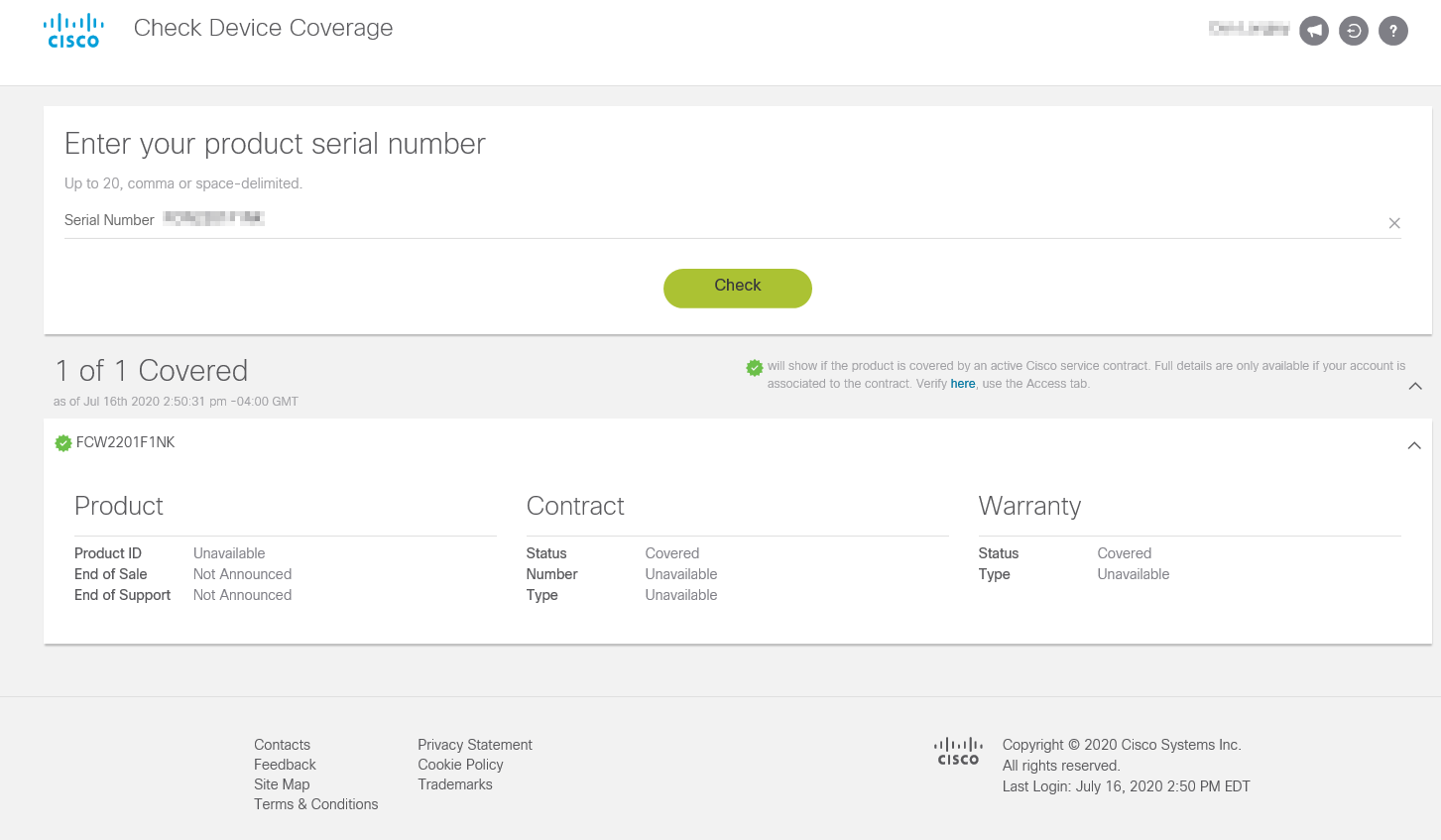The web page features a clean, white background. At the top, the Cisco logo is prominently displayed in blue, accompanied by a small icon above it. The header reads "Check Device Coverage." Towards the upper right corner, there are three gray circles, each containing a distinct symbol.

Directly below the header is a wide input field requesting the user to "Enter your product serial number" (up to 20 characters), with the serial number area blurred out. Situated at the bottom of this input field is a green oval button labeled "Check." 

A light gray divider separates this section from the next. The following area is also white and displays a notification stating "1 of 1 Covered," along with a table containing columns for "Product," "Product ID," "End of Sale," "End of Support," "Contract," and "Warranty."

At the bottom of the page, a gray footer features links listed as "Contact," "Feedback," "Site Map," "Terms and Conditions," "Privacy Statement," "Cookie Policy," and "Trademarks." To the right, it includes the Cisco logo alongside the text: "© 2020 Cisco Systems, Inc. All rights reserved." Additionally, it notes the last login date and time as July 16, 2020, at 2:50 PM Central Daylight Time.